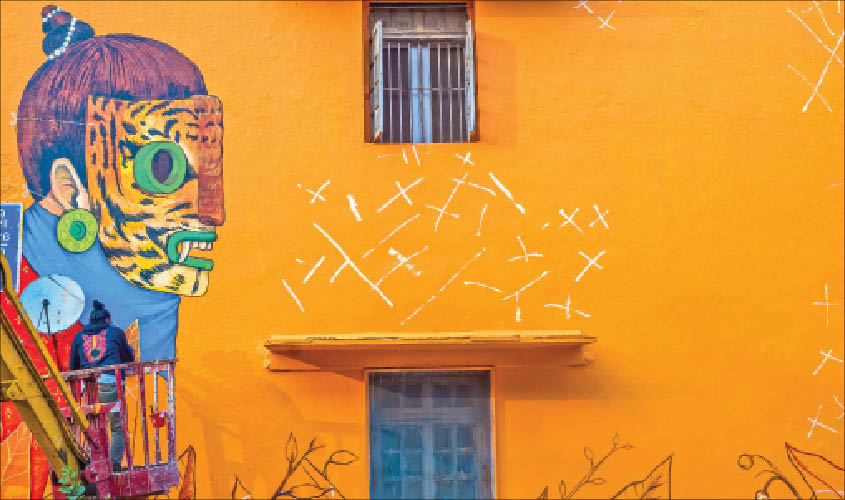The image captures a vibrant outdoor scene featuring a large mural on the bright orange facade of a building. The building resembles the color of an orange fruit with a window at the top, secured with bars, and a door at the bottom topped with an orange awning. The mural, located on the left side of the wall, depicts a person wearing a tiger-print mask with striking green eyes, green lips, and an open mouth revealing teeth and a fang. The figure has brownish hair styled in a bun adorned with white pearls and is also adorned with green disc-like earrings. They are dressed in a blue and red top. Additionally, the mural features illustrations of leaves and numerous white marks near the bottom. During the day, an artist is seen in a cherry picker or crane, actively painting the mural, adding an element of dynamic creativity to the scene.